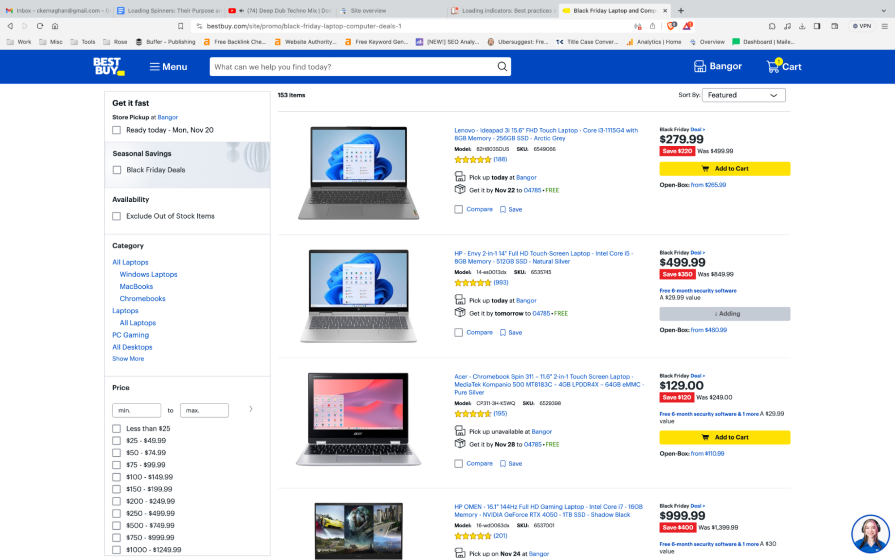Caption: 

The Best Buy web page prominently features a variety of laptops showcased down the center of the page, complete with brand names, detailed features, customer ratings, and availability information. Featured brands include Lenovo, HP Envy, Acer, and HP Omen, with prices ranging from $129.99 for the Acer Chromebook to $999.99 for the high-end HP Omen. The page provides options for pickup locations, delivery times, and even savings on open-box models. Users can easily add items to their cart and see potential savings. On the left sidebar, you have the ability to filter results by price, seasonal promotions like Black Friday deals, and categories such as PC Gaming or All Desktops. A "Show More" option expands further choices. At the top, the classic blue Best Buy header houses a search bar for specific queries, allowing users to navigate quickly to their desired products.